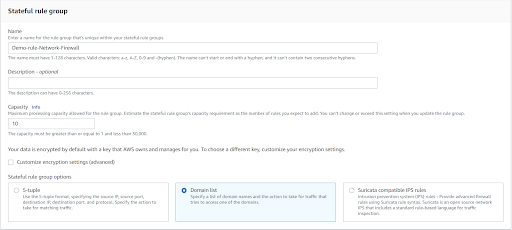This image portrays a detailed panoramic view of a website interface featuring a form with exceptionally small text. The container of the form is encased in a thin gray outline, giving it a clean, structured appearance. 

At the very top of the image, there is a long, thin gray bar. In the far-left corner, in black letters, it appears to say "Dateful Rule Group", although the text is not entirely clear.

Beneath this header, the form begins with a white background. The first section prompts for a name, marked with the word "Name" followed by an instruction to "Enter a name". Below this, there is a faintly readable text box with the placeholder text "Demo-Rule-Network-Firewall".

Next, there is a section labeled "Description (Optional)" with a large empty text box below it. Unfortunately, further explanatory text appears too small to decipher, but there seems to be a character limit mentioned, with a visible number in the thousands, followed by the word "Characters".

Following this, there is a segment titled "Capacity Info". This part includes a brief string of text too small to interpret, followed by a shorter text box defaulted with the number "10". Subtle gray text beneath this box seems to state information regarding capacity limits, containing words like "The Capacity", "Greater than One", and "From 50,000".

Further down, slightly larger text reads: "Your data is encrypted by default with a key that...", though the remainder of the sentence is indistinguishable. The subsequent line says, "To choose a different key, customize your encryption settings."

Directly below this message is a checkbox with accompanying black text that is again, too minute to recognize. Then, there's a label mentioning a "Group Option", followed by three checkboxes. The second checkbox is selected, highlighted in blue with a red dot in the center, though the text adjacent to these options remains unreadable due to its minuscule size.

The form is densely packed with information, but the text is so tiny that full comprehension is hindered. Overall, the image conveys a complex web form filled with various fields and settings, predominantly focused on rule or network management, with a strong emphasis on encryption and capacity limits.